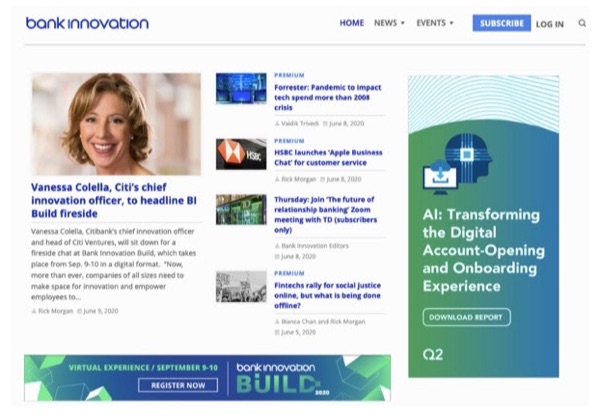**Caption:**

The image depicts a webpage from 'Bank Innovation'. In the top left corner, the text "Bank Innovation" is prominently displayed in blue. The top right section features five tabs for navigation: *Home*, *News*, and *Event*, followed by two buttons, *Subscribe* and *Log In*, as well as a search button. Both the *Home* and *Subscribe* tabs are highlighted in blue, indicating active selection, while the other tabs are in grey.

On the main page's left side, there is a picture of a woman. Below her image, a blue text announces, "Vanessa Corlella, Citibank's Chief Innovation Officer, to headline BI Build Fireside." This is followed by a black text paragraph that provides additional details: "Vanessa Corlella, Citibank's Chief Innovation Officer and Head of Citibank Ventures, will sit down for a faster chat at Bank Innovation Build which takes place from September 9 to 10 in a digital format. Right now, more than ever, companies of all sizes need to make space for innovation and empowerment of employees to lend their techs."

On the webpage's right side, several premium articles and reports are listed:
- "Forester: Pandemic to Impact Tech Spend More Than 2008 Crisis"
- "HSBC Launches April Business Chat for Customer Service"
- "Join the Future of Relationship Banking Zoom Meeting with TD, Subscribers Only"
- "Find Tech Rally for Social Justice Online but What is Being Done Offline"

Additionally, there is an advertisement on the right side, which promotes a report titled "AI Transforming the Digital Account Opening and Onboarding Experience." The advertisement is styled with white text on a green background.